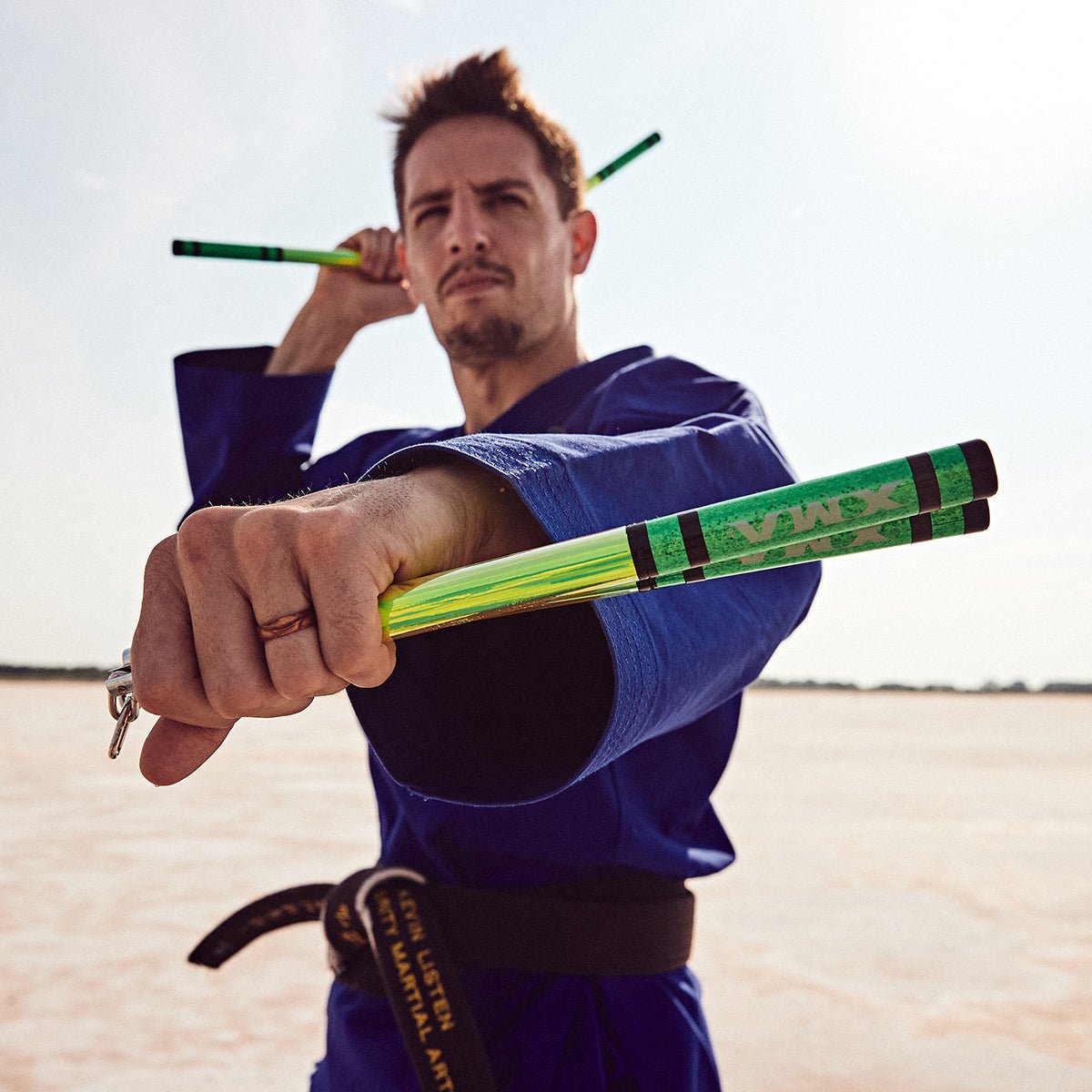In this photograph, a tall, fit man with short, gelled-up brown hair, a goatee, and brown bushy eyebrows strikes a martial arts pose on a beach with water in the background. He is dressed in a dark blue karate suit (kata) and wears a black belt around his waist, which is adorned with yellow stitched text stating "Listen Martial Arts." The man, wearing a brassy copper-colored ring on his finger, holds a pair of bright green nunchucks in each hand. One arm is raised behind his head while the other is extended forward, both nunchucks gleaming with green glitter and marked with the text "VMX" on black bands positioned on the center and at the edges. His facial expression is serious, completing his composed yet dynamic stance.